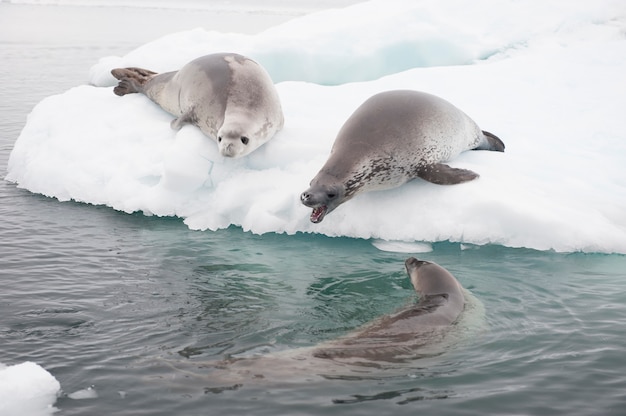In this richly detailed photograph set in what appears to be a natural Arctic or Antarctic habitat, three seals are captured interacting on and around a floating ice floe. The ice is a bright white, contrasting dramatically with the dark blue-gray waters surrounding it. Two seals are perched close together on the ice, with one seal’s mouth ominously open as if barking or leering towards the third seal in the water. This seal in the water, located towards the right side of the image, has its head protruding into view, looking up at its companions. The seal on the left of the ice is slightly lighter in color, blending in with the snowy backdrop, accentuated by patches of gray on its nose and above its eyes, and black flippers tinged with gray. Meanwhile, the seal on the right, which appears darker and more mottled, has more pronounced gray spots and darker flippers. The scene suggests a dynamic interaction, possibly a moment of tension or play in the seals' natural icy habitat.